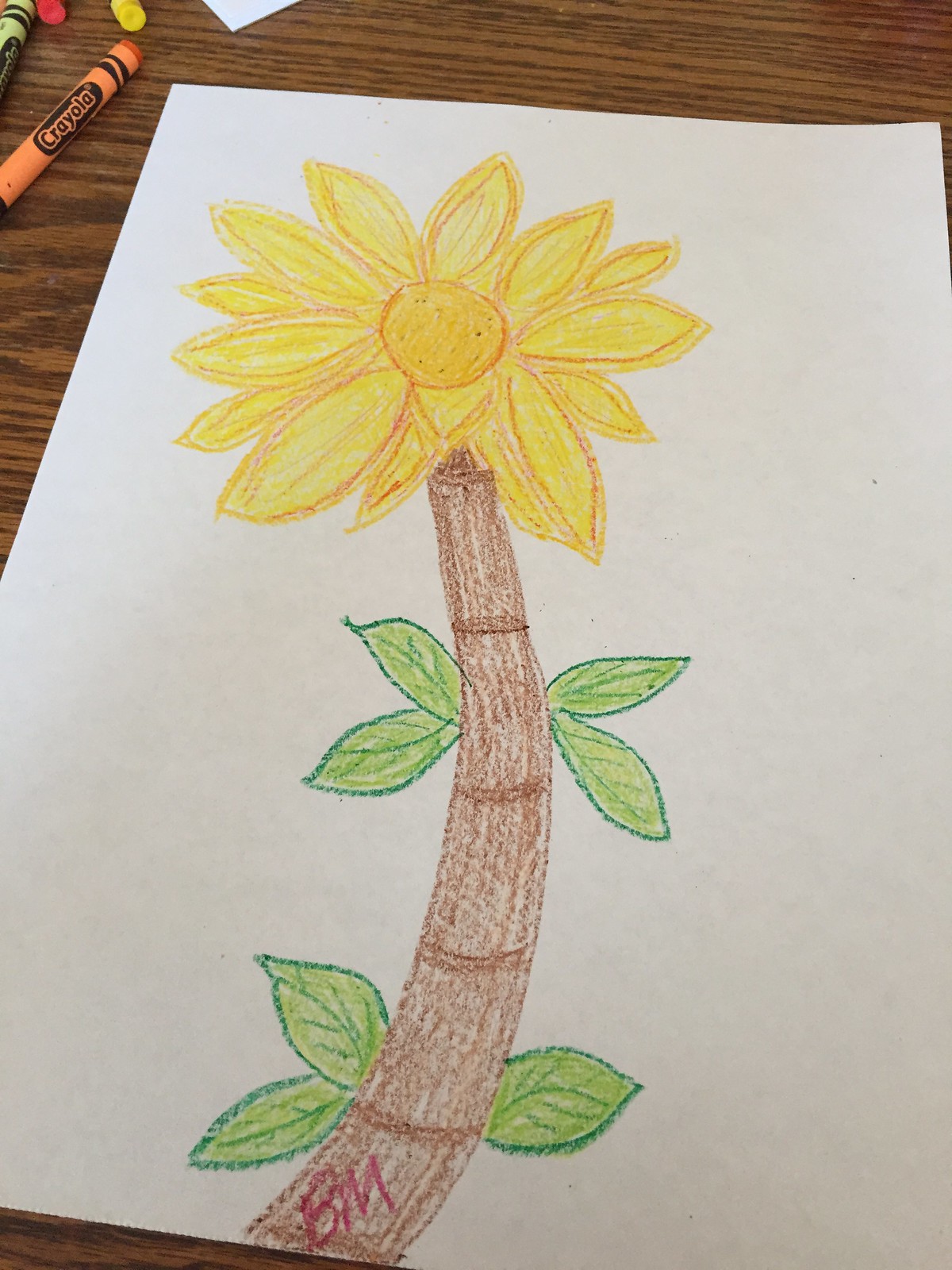This photo captures a charming hand-drawn sketch on a piece of white paper, crafted with crayons. The focal point of the sketch is a vibrant flower, featuring a yellow head with multiple layers of yellow petals, artistically outlined in brown. The central portion of the flower is dotted with speckle marks, adding texture and depth. The flower is anchored by a brown stem, which has horizontal marks running along its length, resembling a reed. Flanking the stem are several green leaves, adding a splash of color to either side of the sketch. In the corner of the image, a few Crayola crayons are casually laid on the table, hinting at the creative tools used to bring this delightful drawing to life.